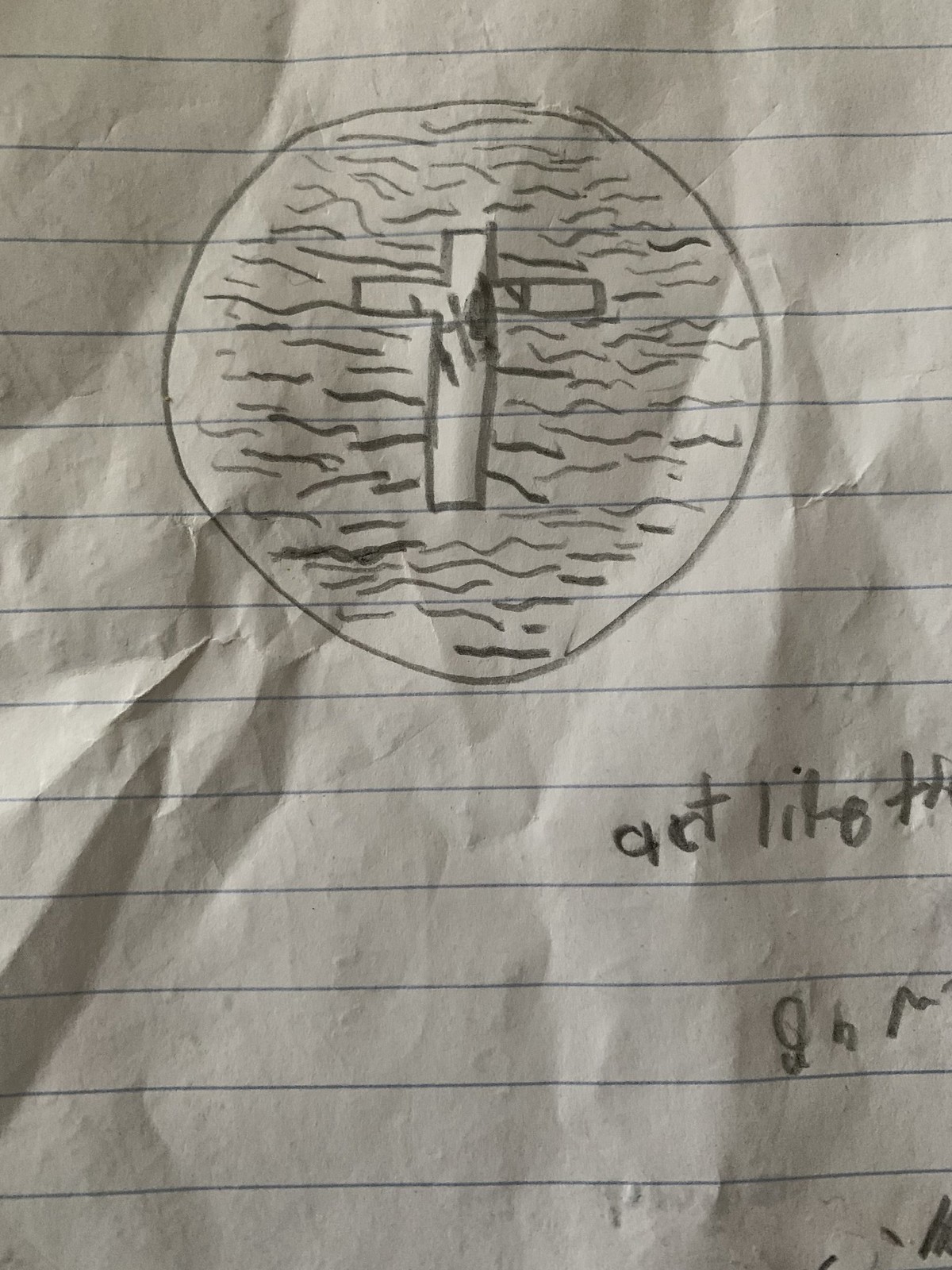This detailed image portrays a close-up of a piece of lined paper, slightly crumpled, with a hand-drawn design in pencil. Central to the design is a Christian cross, featuring a horizontal bar near the top intersecting a slightly longer vertical bar. Unreadable black markings or letters, potentially forming a shape resembling an 'H,' are present on the cross, but it's ambiguous whether they are intentional letters or coincidental lines.

Encircling the cross is a circle filled with wavy patterns reminiscent of waves, also rendered in pencil. The lined paper sports faint blue horizontal lines, typical of notebook paper, and shows imprints from writing on the underlying page. At the bottom right of the image, partially legible writing appears to spell out "A-C-T," though the remainder of the text is indecipherable. The overall composition suggests a blend of haphazard scribbling and deliberate drawing, adding an enigmatic quality to the artwork.